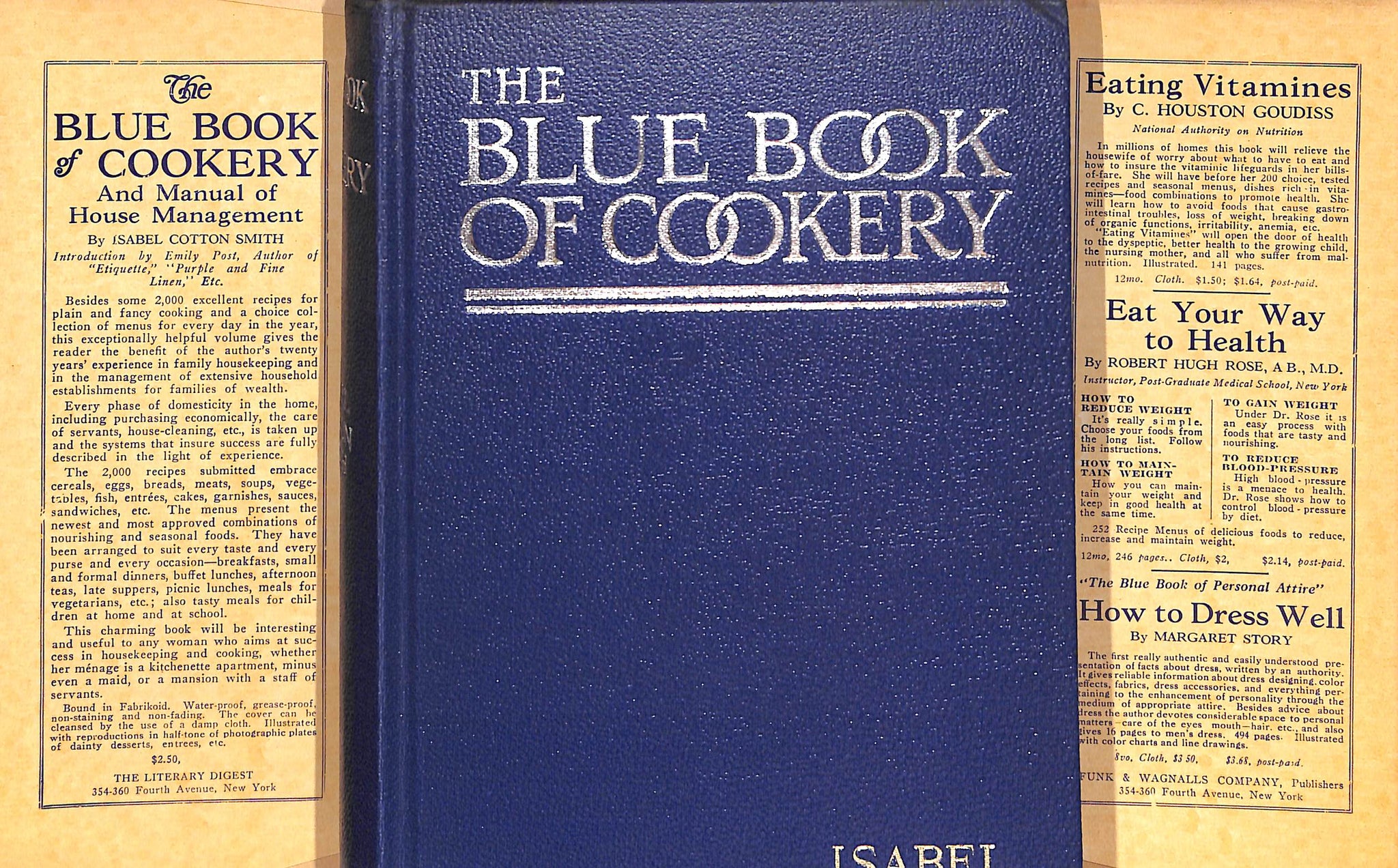The image features a vintage hardcover book at its center, entitled "The Blue Book of Cookery" in silver embossed letters on a solid royal blue cover. At the bottom right of the cover, partially visible text reads "Isabel," which is possibly the author’s name. Flanking the book are two aged, yellowed pages. 

On the left page, the text begins with "The Blue Book of Cookery and Manual of House Management by Isabel Cotton Smith." It presents a detailed description of the book, highlighting its 2,000 recipes for plain and fancy cooking, and various menus suitable for every occasion. The description emphasizes the author's 20 years of experience in family housekeeping and household management. It also mentions that the book covers exhaustive aspects of domestic management such as purchasing economically, caring for servants, and house cleaning, and offers assurances that it will benefit any woman aiming for success in housekeeping, regardless of her household size or means. The page concludes with the publication details: "The Literary Digest, 354-360 4th Avenue, New York," and a price of $2.50.

The page on the right features headlines and brief articles. The first headline reads "Eating Vitamins" by C. Houston Goudis. The second, "Eat Your Way to Health" by Robert Hugh Rose, A.B., M.D., is followed by a substantial article. The final headline is "How to Dress Well" by Margaret Story, beneath which is text that is harder to read. 

The overall composition of the image conveys a rich historical and domestic instructional focus with an emphasis on practical household management and cooking expertise.